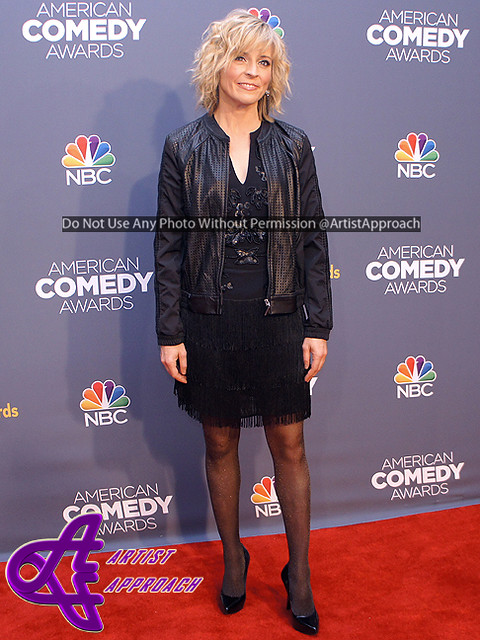The image depicts a middle-aged, blonde actress standing on a red carpet at an NBC event, specifically the American Comedy Awards. She is dressed in a stylish, all-black ensemble featuring a leather jacket, a black top, a knee-length black skirt with frills, knee-high stockings, and high-heeled shoes. The backdrop behind her repeats the phrases "American Comedy Awards" and "NBC," featuring the iconic multi-colored peacock logo in shades of yellow, orange, red, purple, blue, and green. The actress is smiling broadly, showing her top row of teeth, and has her arms resting by her side. In the bottom left corner of the image, there is a purple graphic logo resembling two intertwined 'A's with the text "Artist Approach" beside it. Additionally, a watermark across the photo reads, "Do Not Use Any Photo Without Permission," along with the social media handle "Artist Approach."